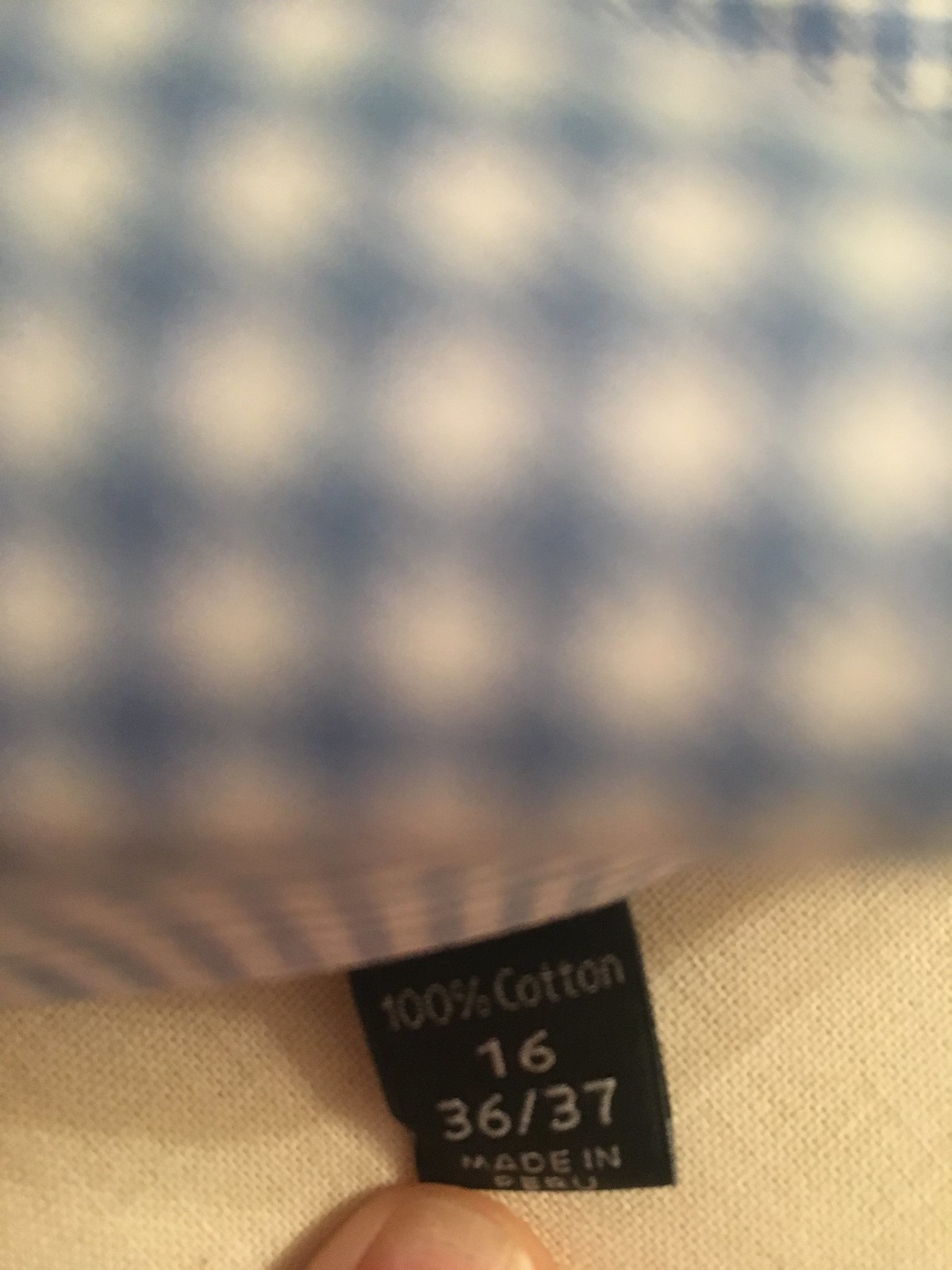This close-up color photograph showcases the tag on a checkered shirt, primarily focusing on the tag itself while the shirt is notably blurred. The shirt features a blue and white checkered pattern, giving it a tic-tac-toe-like appearance. The tag is black with white and gray lettering, clearly stating "100% cotton" at the top. Below this, it indicates the size "16," followed by measurements "36 by 37," and finally mentions that the garment is "Made in Peru." The image also captures a person's thumb and partial thumbnail holding the tag, emphasizing its position for the photograph. The inner side of the garment appears as a white woven material, contrasting with the blue and white checkered fabric. The shirt’s checkered pattern occupies the top part of the image in a blurred state, while the tag and the assisting finger dominate the bottom half.